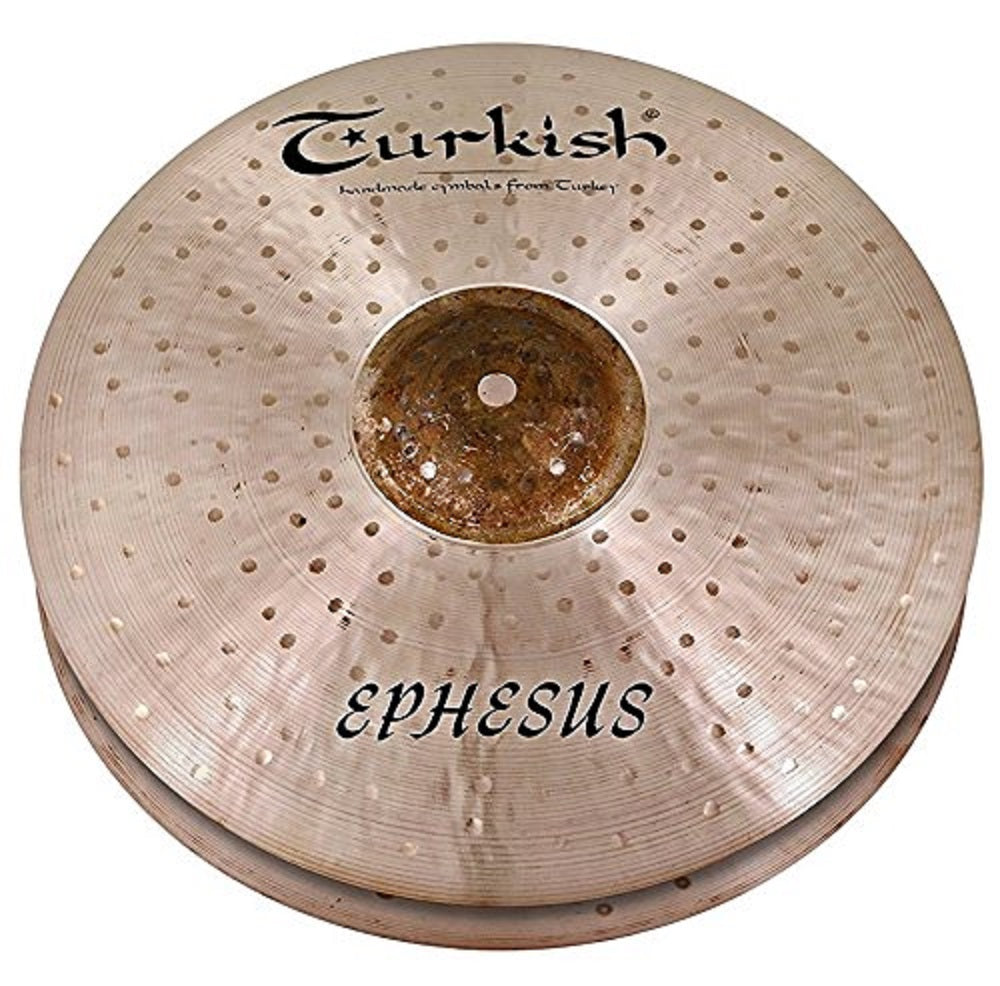The image depicts a worn and weathered circular silver metal object, possibly a disc brake or a cymbal. The surface is covered in several small, circular dimples and indentations, some of which are dirty, giving it a well-used appearance. Prominently, the object features a heavily rusted area in the center, making up about one-fourth of its diameter. Near the top, in large black lettering, it reads "Turkish," with a star behind the 'T'. Below this, there is smaller, hard-to-read text that likely says "handmade symbols from Turkey." Additionally, at the bottom of the object, the word "Ephesus" is inscribed in all capital letters. The overall condition, including the rust and numerous dings, suggests the object has been exposed to the elements for an extended period.